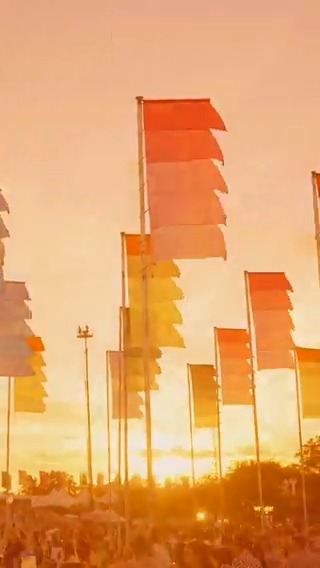In a scene drenched in golden, peachy sunlight, multiple vertical flagpoles rise above a large, indistinct crowd, evoking the atmosphere of a sun-saturated festival or desert fairground. The flags, resembling pride banners, feature vibrant colors arranged in gradients from dark red to light pink, orange to yellow, and mauve. Each banner is stiffened outward by horizontal poles and flutters slightly in the bright, hazy light. The overexposure of the image lends a strong yellow and orange hue, obscuring finer details but revealing a glimpse of tents and people beneath the tree line, along with a weather vane and possible antenna adding to the ambiance above. Despite the crowd's presence and festival feel, the intense sunlight makes specific details hard to discern.